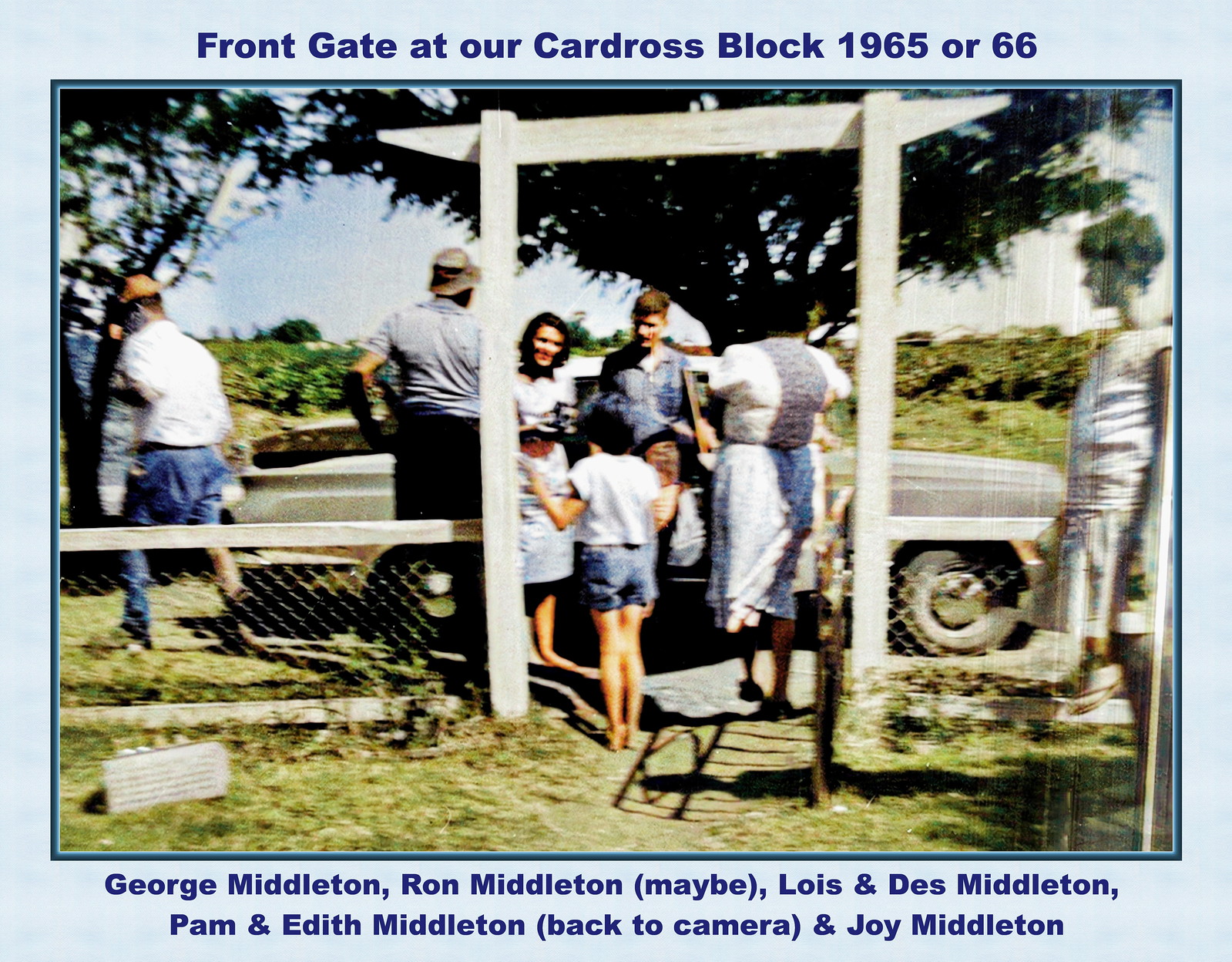This vintage photograph from 1965 or 1966 captures a nostalgic moment of a family gathered in the front yard of their home. At the center of the scene, an old 1950s or 1960s automobile is parked near a wooden gate, which leads to the yard. A man and a woman stand by the car, while another woman and a child are positioned before them. Additional family members mill around, contributing to the lively atmosphere. The child is notably standing under a tall white wood post, with a fence lined with chicken wire enclosing the space on both sides. A large leafy tree provides shade, and in the background, expansive corn fields stretch out, adding a rural charm to the setting. The top of the photograph is labeled with the caption "front gate at our car dress block, 1965 or 66," and the bottom includes a list of the people present, ensuring everyone is recognized in this cherished family memory.